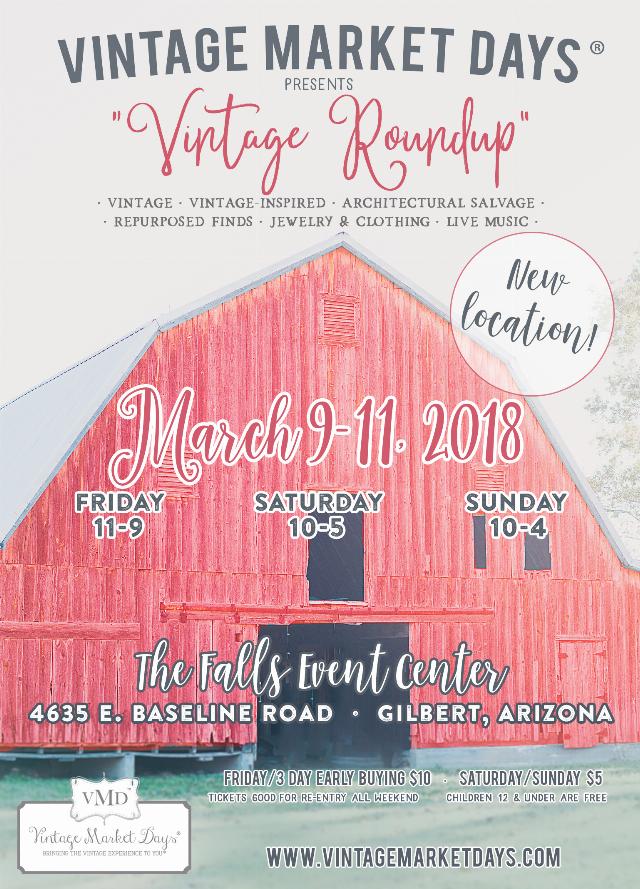The image is an advertisement for the Falls Event Center, located in Gilbert, Arizona, showcasing the Vintage Market Days event titled "Vintage Roundup." The background features a painting of a large red barn with a white roof, set against a grassy foreground and a white sky. The advertisement highlights that the event will take place from March 9th to 11th, 2018, with operating hours of Friday from 11 AM to 9 PM, Saturday from 10 AM to 5 PM, and Sunday from 10 AM to 4 PM. Bold red and black text, with some titles in cursive, announces various attractions including vintage, vintage-inspired, architectural salvage, repurposed finds, jewelry, and clothing, along with live music. Additional details mention a special early buying opportunity on Friday for $10, with tickets valid for re-entry throughout the weekend, while general admission for Saturday and Sunday is $5, and children 12 and under enter for free. The event’s location is specified as 4635 East Baseline Road, Gilbert, Arizona. Further information can be accessed at www.VintageMarketDays.com.